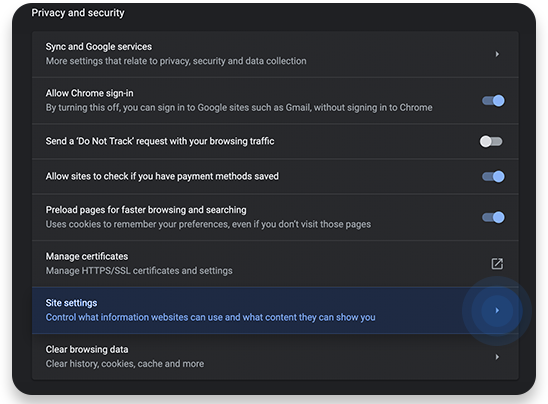The screenshot displays a mobile device screen, which could be a smartphone or tablet, most likely running either iOS or Android, showing a section of browser settings related to privacy and security. The background is black, and the text is predominantly white. 

In the upper left corner, the heading "Privacy and Security" is displayed, under which "Sync and Google services" is listed. Below this section, in gray, there is an option labeled "More settings related to privacy, security, and data collection" accompanied by a rightward-pointing arrow.

Underneath this, a highlighted option reads "While Chrome is signed in," with a subordinate explanation: "By turning this setting off, you can sign into Google sites such as Gmail without signing into Chrome." 

Further down, another setting in blue titled "Send 'Do Not Track' request with your browser traffic" is shown as turned off. 

Following this, the option "Allow sites to check if you have payment methods saved" is displayed with a blue checkmark indicating it is enabled. 

Additional settings listed include "Preload pages for faster browsing and searching," displayed in white, and "Use cookies to remember details of your visits," which is turned on.

Two more options are "Manage certificates" and "Manage HTTPS," each accompanied by a rightward-pointing arrow.

A blue-highlighted section titled "Site settings" informs the user about controlling the information that websites can use and show. 

Finally, a section titled "Clear browsing history" is highlighted in white on a black background, with the subtext "Clear history, cookies, cache, and more" presented in gray below it.

This detailed narrative captures all the elements visible in the settings screenshot.